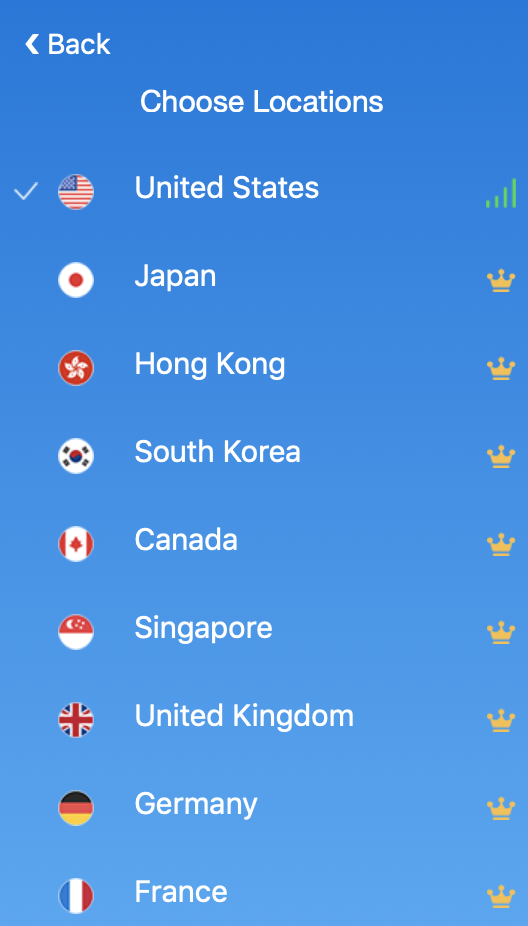The image appears to be a screenshot taken from a mobile phone or a vertically held tablet. The vibrant blue background typical of many interfaces is immediately noticeable. At the top of the screen, there is a back button. Centered prominently below this, the text "Choose Locations" is displayed, with both 'C' and 'L' capitalized. 

A list of countries follows: United States, Japan, Hong Kong, South Korea, Canada, Singapore, United Kingdom, Germany, and France. Each country is represented with a small round icon displaying a portion of its respective national flag. The United States has a checkmark to the left of its flag and a signal strength bar to the right, indicating it is the currently selected location. For all other countries, a yellow crown symbol is placed to the right of their flags, possibly indicating premium or VIP status.